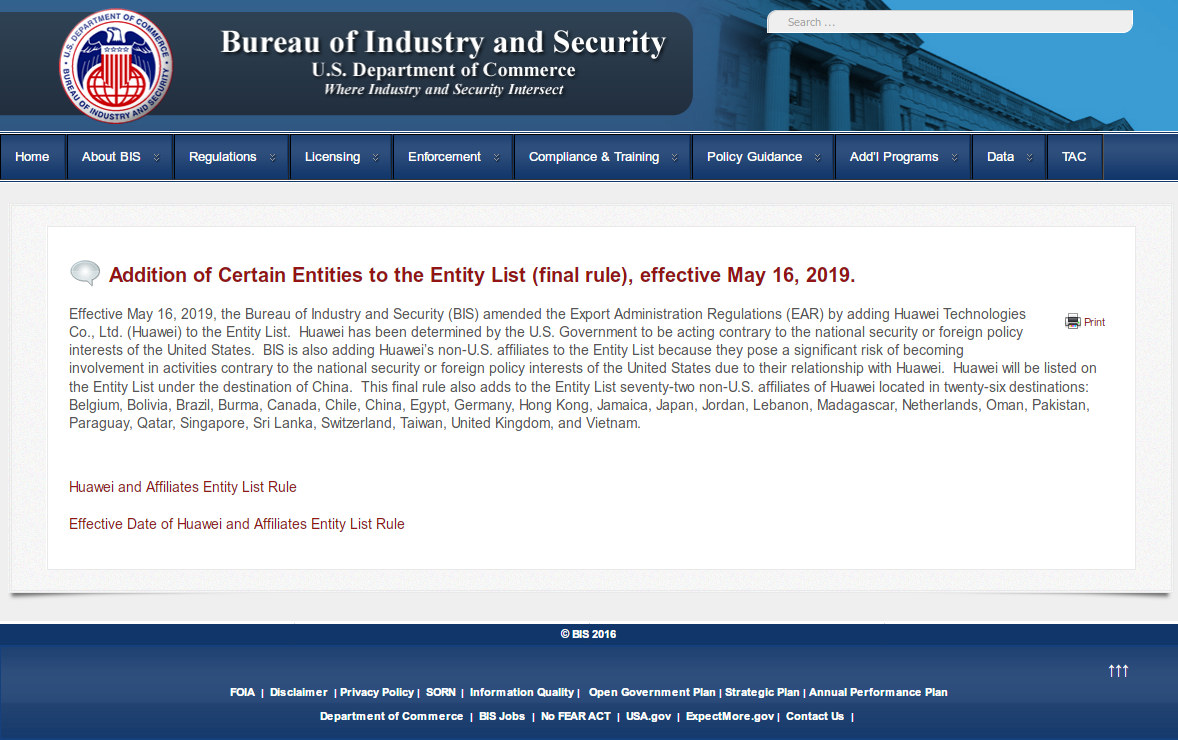The image features a dark blue border in the top left corner, gradually lightening to a lighter blue shade towards the right. On the left side, there is an official government logo depicting an eagle and a globe, adjacent to the text "Bureau of Industry and Security, U.S. Department of Commerce: Where Industry and Security Intersect." To the right of the logo is an image of a grand building that resembles a courthouse, complete with tall, imposing columns. On the upper right side of the image, there is a search bar. Below the search bar, the image displays several navigation tabs labeled Home, About BIS, Registration, Licensing, Enforcement, Compliance and Training, Policy Guidance, Programs, and TAC. Beneath these tabs, a prominent red text announcement reads: "Addition of Certain Entities to the Entity List. Final Rule, effective May 16, 2019."